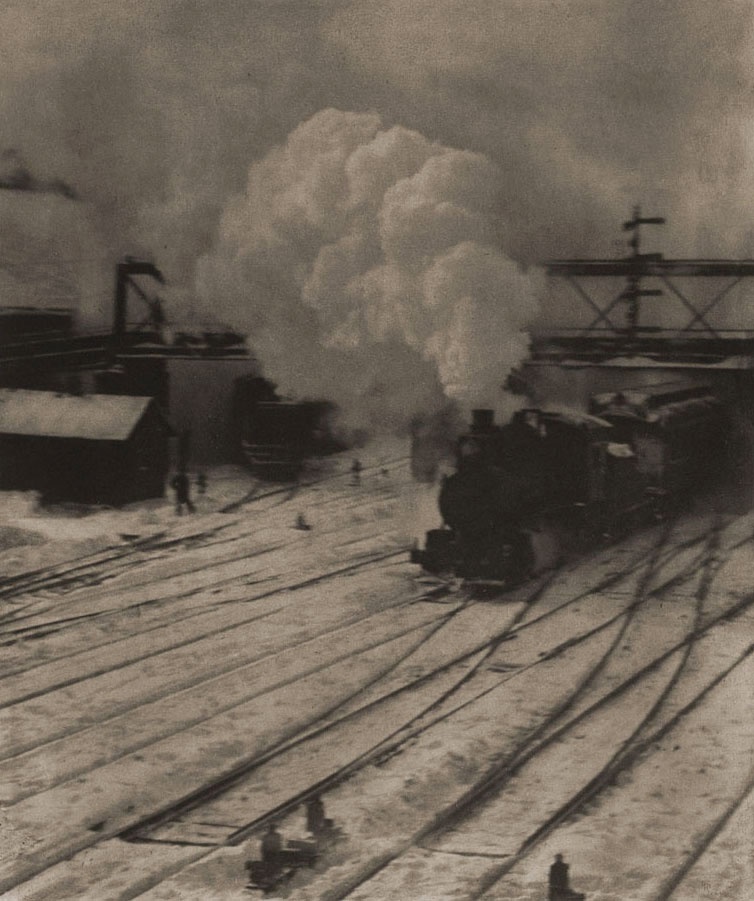This vintage black-and-white photograph captures a bustling winter scene at a train yard. At the center of the image, a steam locomotive, billowing a thick cloud of white smoke, moves along a set of multiple train tracks that crisscross the ground in various directions. The grainy image, likely taken from a high vantage point, features a main train passing underneath an industrial bridge or trellis. To the upper left, a large gas tank is visible along with electrical and telephone wires stretching across the backdrop. The dated and overcast atmosphere is accentuated by the presence of silhouetted figures, including two prominent ones on the tracks, possibly workers using shovels. More workers and individuals are seen on the side of the tracks and around a nearby station, which likely serves as a ticket office and rest area for train personnel. The overall composition, including people, the old station, and the intricate network of tracks, paints a vivid picture of a historical moment in railway history.